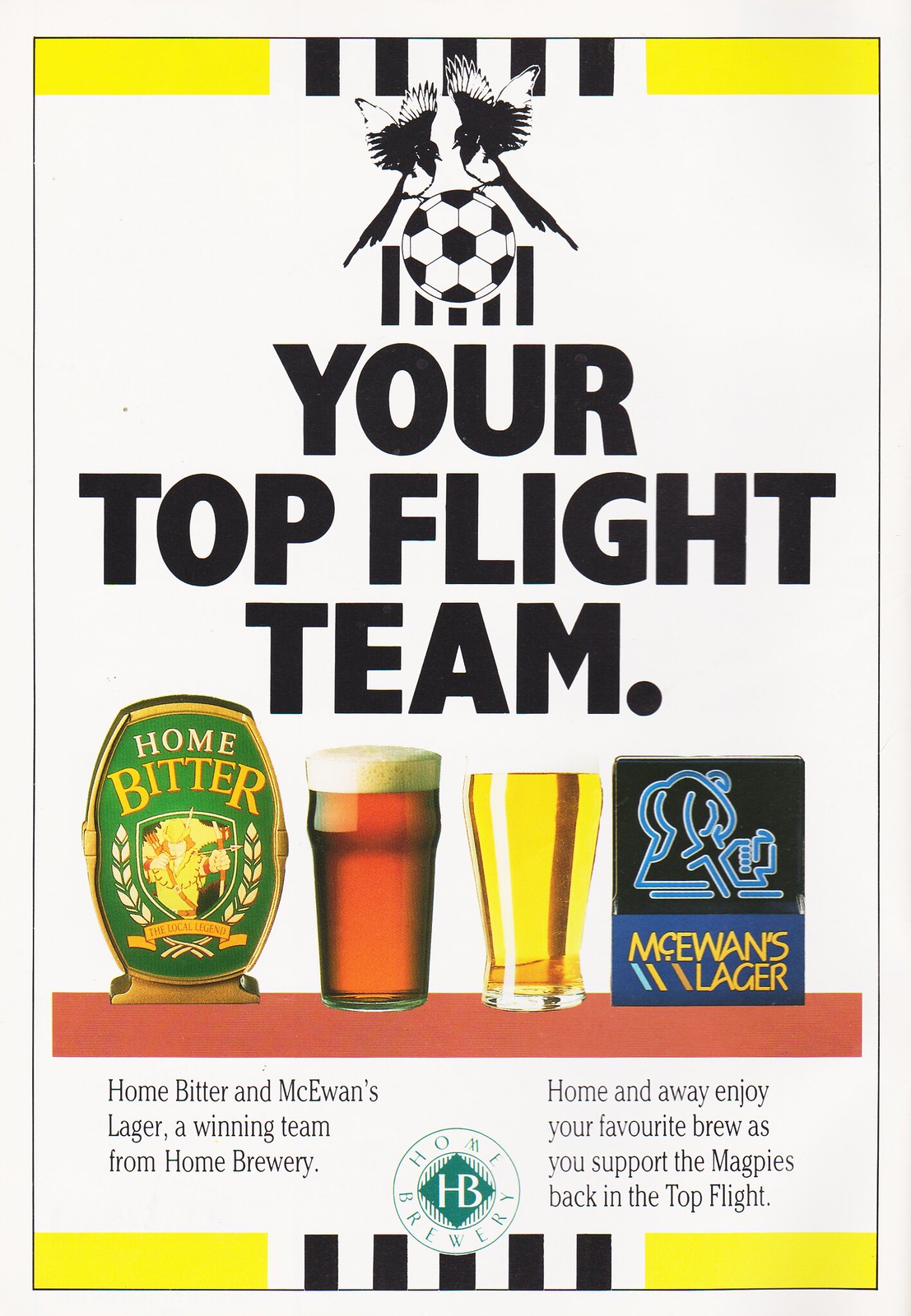The image is an advertisement flyer with a white background, accented by yellow stripes at the top and bottom. At the top center, there is an image of two birds sitting on a soccer ball. Below the image, in bold, capitalized black letters, are the words "YOUR TOP FLIGHT TEAM." Beneath this text are images of several different beers. One prominently features a light ale and a dark ale, labeled as Home Bitter and McEwan's Lager. The darker beer is in a cup, while the brighter yellow beer is in a glass. Following this imagery, there is a red border framing the bottom section. Within this border, a text block states: "Home Bitter and McEwan's Lager: a winning team from Home Brewery. Home and away, enjoy your favorite brew as you support the Magpies back in the top flight."